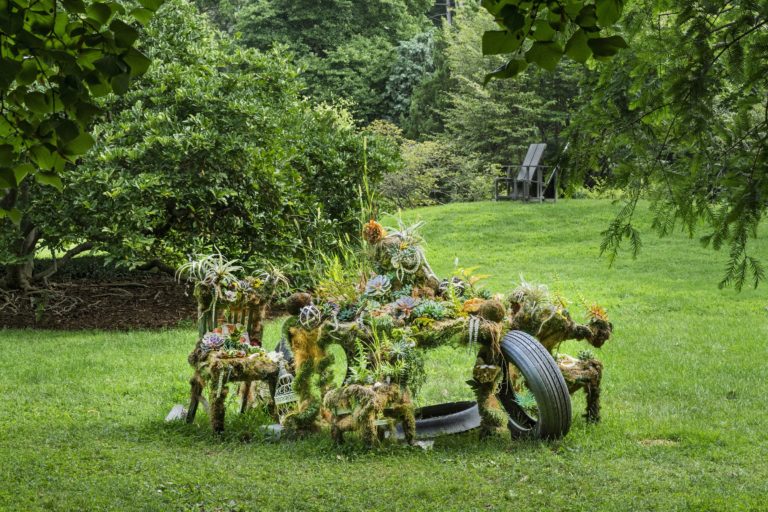In the center of a well-maintained, bright green lawn, the image showcases an artistic outdoor installation, likely in someone's yard or a park. The setting is illuminated by daytime light, revealing a background dense with various trees, including some with broad leaves and others, like pines. The installation itself is a creative assembly of discarded objects, masterfully draped in moss, flowers, and other greenery. Within this earthy display, an old automobile tire and what appears to be wooden desks or benches are prominently featured, partly obscured by the lush vegetation. Among the items, a birdhouse is nestled amidst the plants, while a curious pineapple sits atop the arrangement. The scene suggests an attempt to form a word, potentially "hope" or "home," using these objects and plants. Adding to the eclectic mix, a dark gray wooden chair and possibly a couple of benches are visible in the distance, enhancing the contemplative feel of this imaginative lawn ornament. A small black lawn chair can be seen further back, contributing to the tranquil, yet whimsical atmosphere of this green haven.